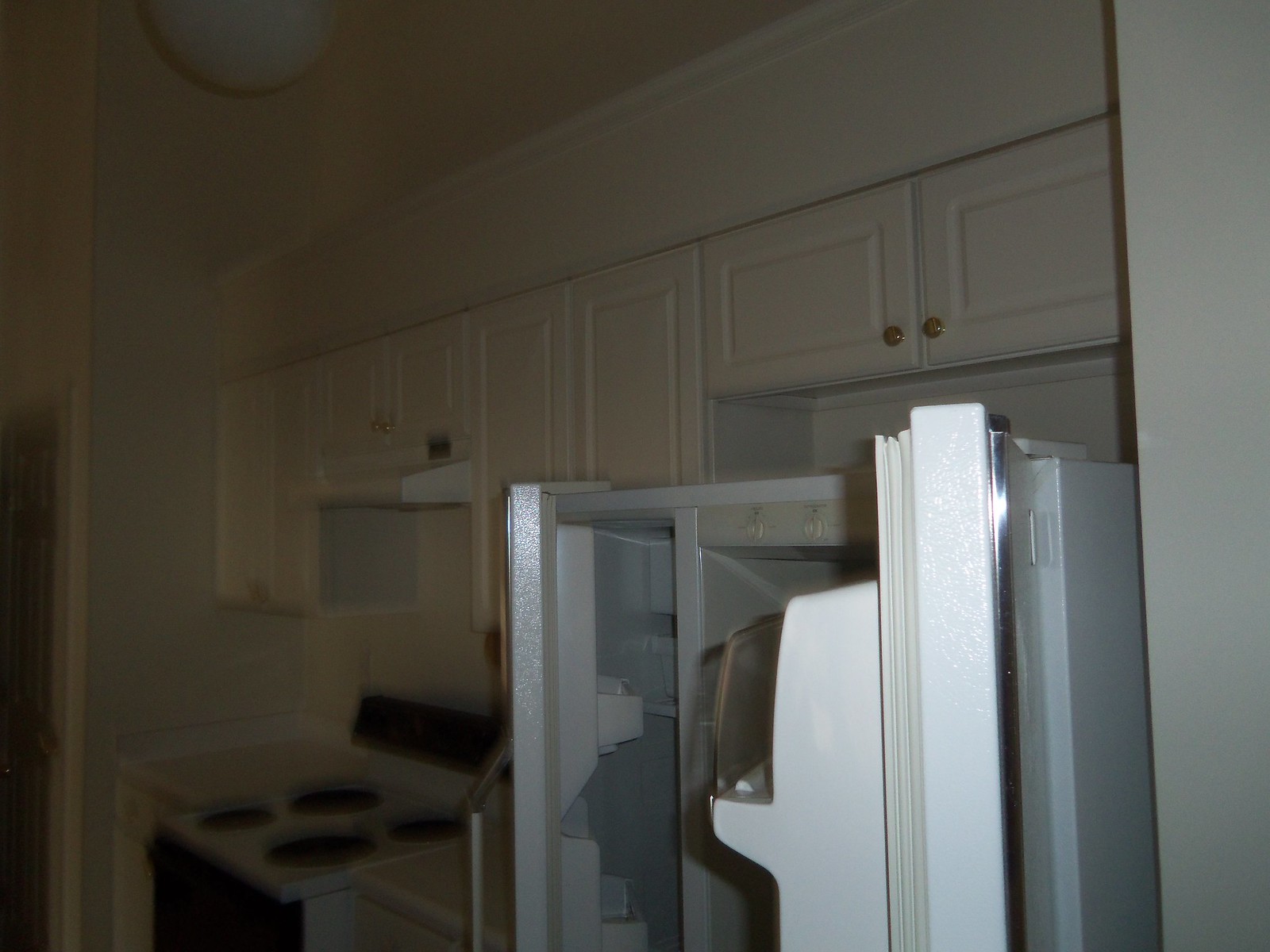The image showcases a dimly lit kitchen with a predominantly white color scheme, characterized by builder-grade white appliances, cabinetry, and walls. The kitchen features a total of eight cabinets—four short and four long—with the short cabinets positioned above the appliances like the stove and fridge, the latter of which has its double doors open, revealing sparse shelving inside. The cabinetry is adorned with gold knobs, enhancing its understated elegance. Centrally hanging from the ceiling is a small dome light. The stove, a classic range stove with black burners and a black front, sits beneath a visible hood. To the left of this setup is a dimly-lit hallway or door, barely distinguishable in the greenwashed ambiance of the image.